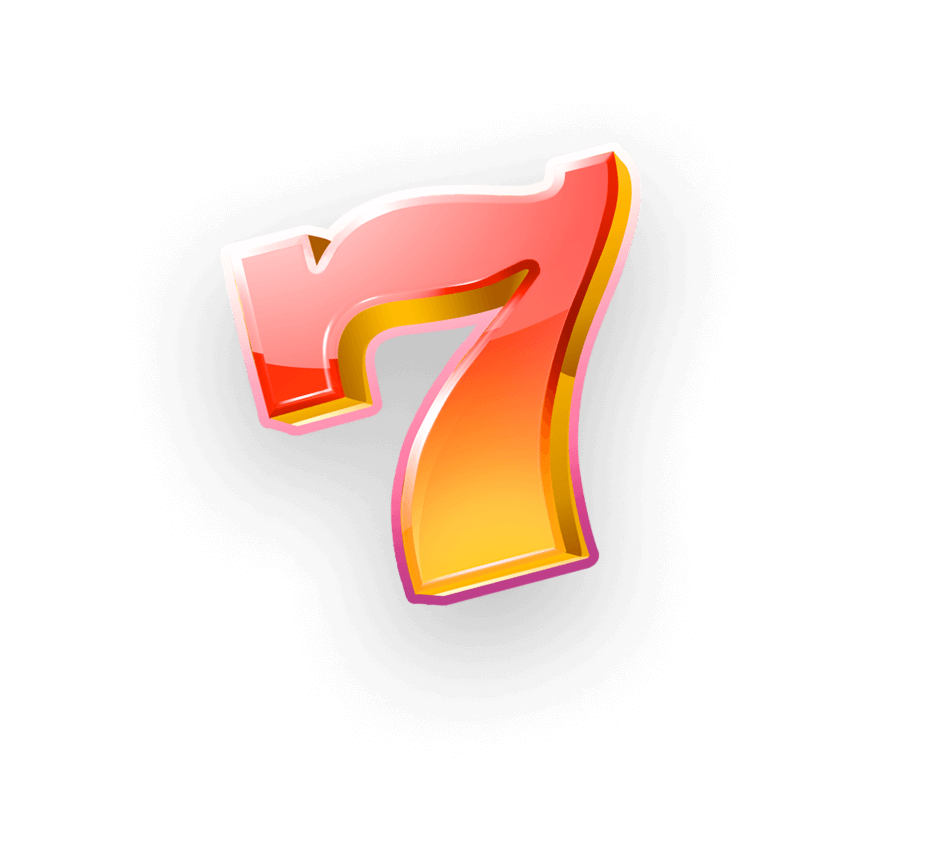The image is a color illustration featuring a stylized numeral seven on a mostly white background that transitions to a light gray or blue toward the center. The seven is embellished with a gradient tint, starting with pink at the top, transitioning through red and orange, and eventually fading to a golden yellow at the bottom. The numeral has a distinctive, almost hammer-like shape that gives it a unique, elegant flow.

This seven is approximately 2 inches tall and 2 inches wide at the top, narrowing to about an inch at the bottom. It is presented in a fancy, script-like font that enhances its three-dimensional effect. The edges of the seven are outlined with a mustard color matching the golden gradient at the bottom, while the outer edges feature a pink outline that deepens toward the base. Additionally, the top of the seven has a white outline, adding to the depiction's layered complexity.

The design includes a drop shadow effect in gold, lending further depth to the number. Surrounding the seven is an ethereal, light white to gray ghosting, which enhances its dramatic and fluctuating appearance. The entire composition is enclosed within a square orientation, accentuating the vivid and intricate design of the stylized numeral seven.